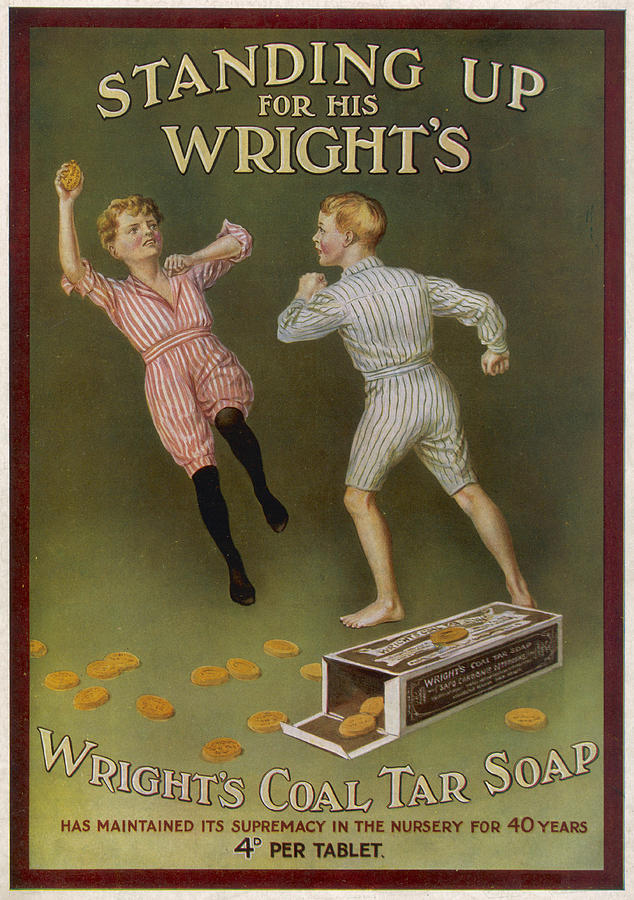An antique poster advertises Wright's Coal Tar Soap with the tagline "Standing up for his rights" featured at the top. The image depicts two red-haired children, a boy and a girl, both in pinstriped pajamas—his being blue with dark stripes and hers red or pink. The boy, appearing charged and defensive, has his arms up as if ready to fend off the girl, who seems poised to throw a bar of soap at him. She wears black stockings to complete her outfit. Scattered around them are bars of soap spilling from an open brown and white packaging. At the bottom, the poster proclaims in white text, "Wright's Coal Tar Soap," followed by the statement in red, "Has maintained its supremacy in the nursery for 40 years." The cost is listed as "4D per tablet," suggesting an older European currency. The entire scene is enclosed in a brown border, maintaining the vintage aesthetic of the poster.